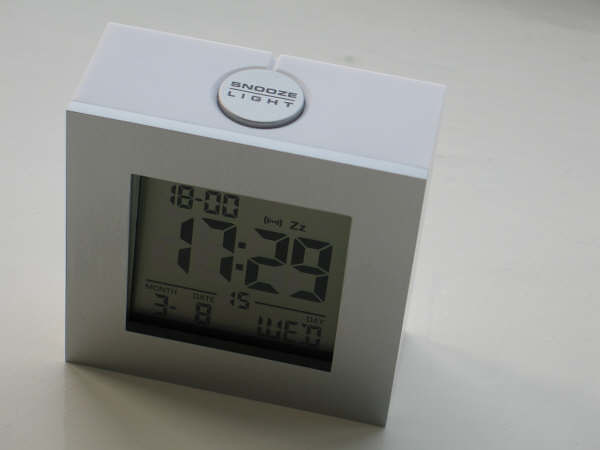This image shows a white digital alarm clock with a cube-like, upright shape standing on a white surface, likely a table. The clock features a slightly indented square display in the center and a prominent circular snooze button on top. The button has a line through it, with "SNOOZE" in capital letters above the line and "LIGHT" spaced out below it. The digital display shows the time as 1729 (5:29 PM) in large black LED numbers against a gray background. At the top of the screen, it also displays the time as 18-00 (6:00 PM). Below the main time display, the clock provides additional information such as the date on the bottom left, showing "month" followed by "3" and another number that suggests the date, possibly "8". On the bottom right, the day of the week is indicated, though it is somewhat obscured by shadows. The clock's sleek, minimalist design is emphasized by its all-white frame and clean lines.